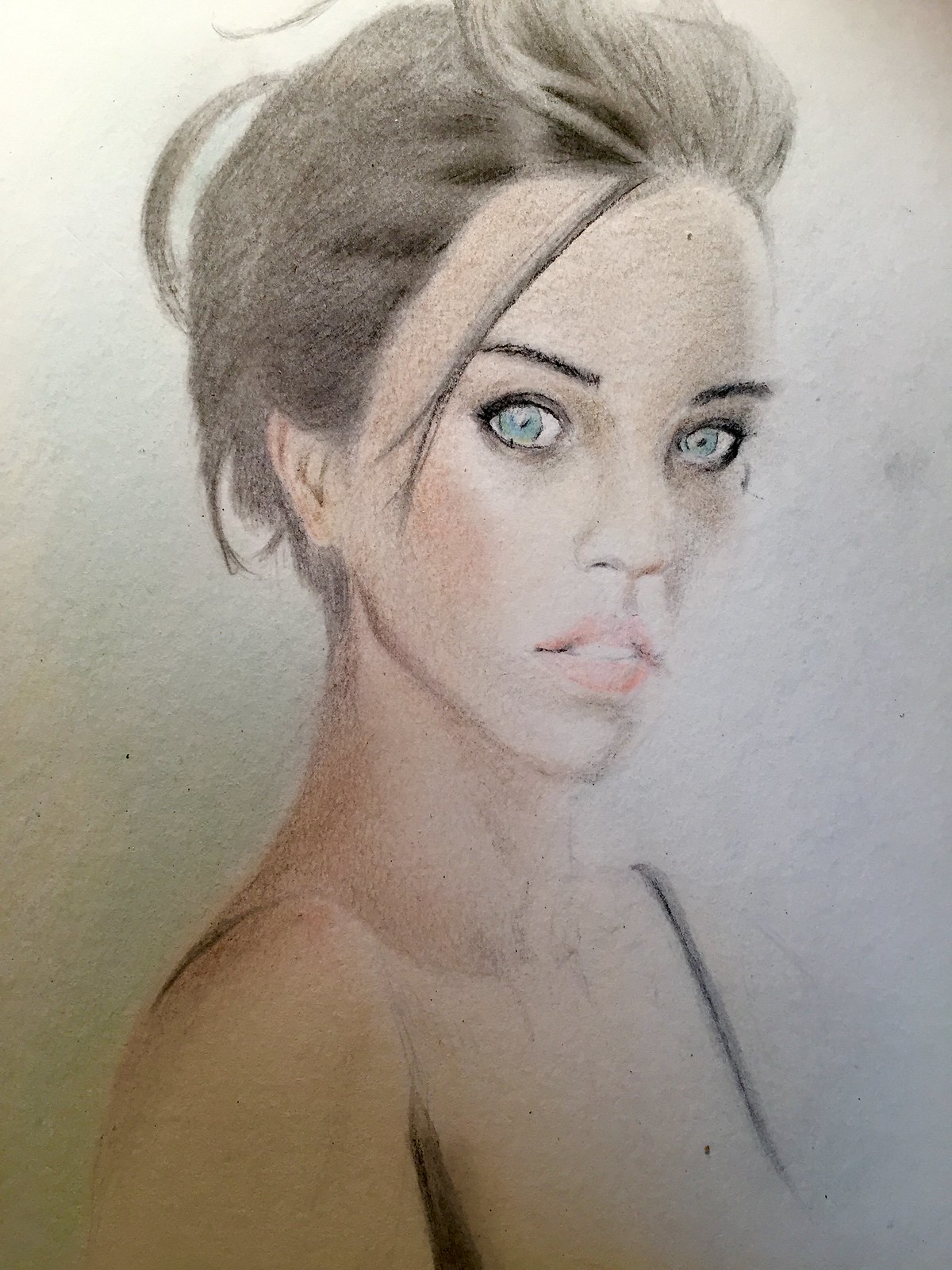This is a detailed portrait of a woman rendered with either pastel or colored pencils. The artwork is rectangular and prominently features the woman's head and upper chest, set against a plain, white background. She has striking black hair, which is styled back with a few strands cascading toward her right eye, delicately grazing her black eyebrows. Her eyes are a vibrant light blue, encircled with what seems to be eye shadow or mascara, accentuating her gaze which is directed straight forward, giving the impression she is looking at the viewer. Her lips are a pinkish color, with the top set of her white teeth slightly visible. She has a long, slender neck and thin shoulders, and she is wearing something black like a halter top or dress, with thin straps visible over her shoulders. The overall composition focuses solely on the woman, with her detailed facial features and minimalist clothing drawing immediate attention.